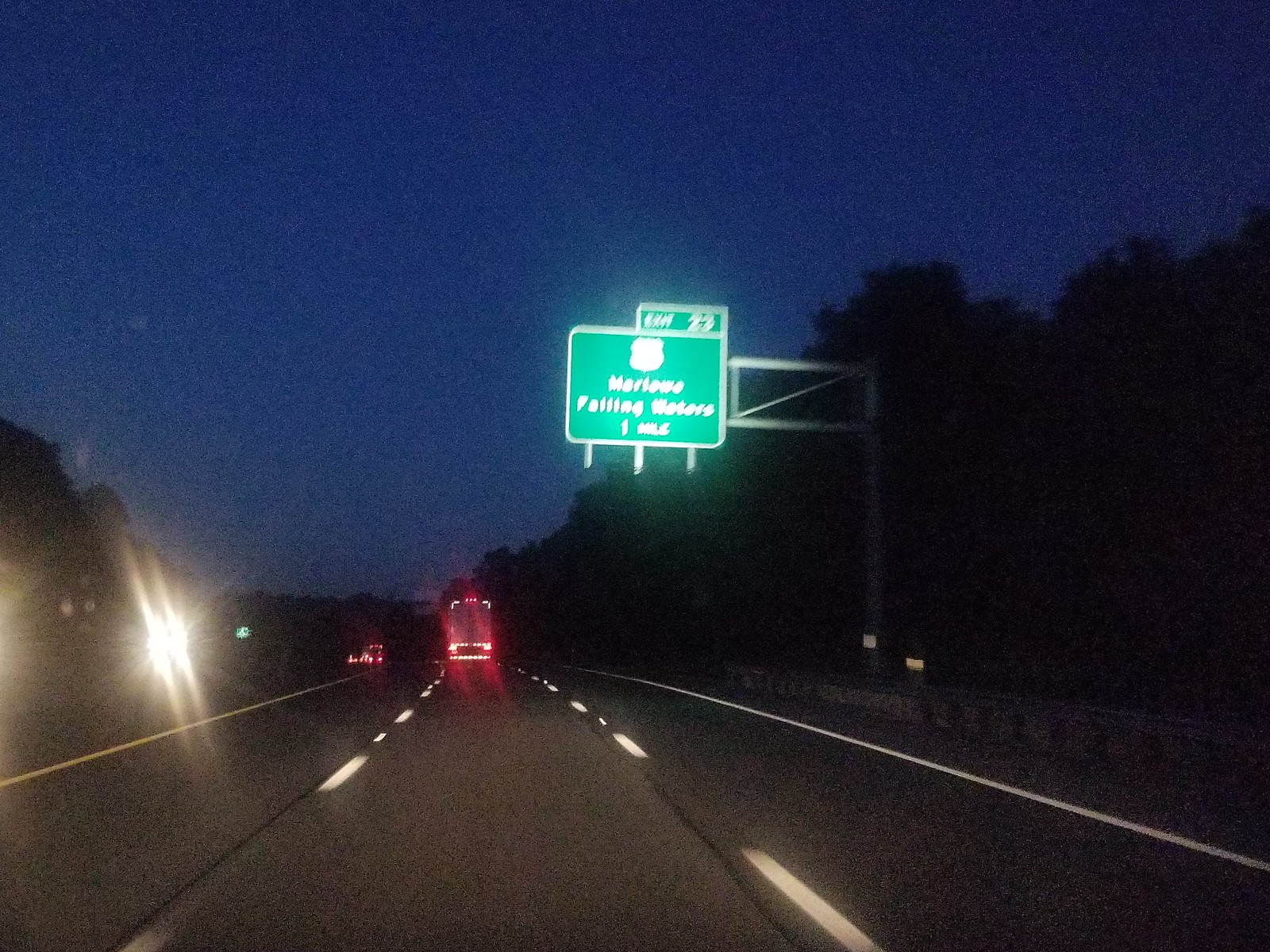A dash cam captures a scene on an interstate highway, likely during early morning or evening hours, as suggested by the dark blue sky devoid of sunlight. The highway is a three-lane stretch, with the camera vehicle traveling in the center lane. Directly ahead is a green exit sign reading "Exit 27," detailing an upcoming exit one mile ahead for a city with an unreadable name and Falling Waters. Appearing prominently in the frame, the sign also features a shield with the road number for the city or state route. Up the road, a noticeable distance away, a tractor trailer with illuminated brake lights is visible, followed by more tractor trailers and vehicles. On the opposite side of the interstate, the headlights of oncoming cars pierce the dim light, offering a contrast to the darkening sky.